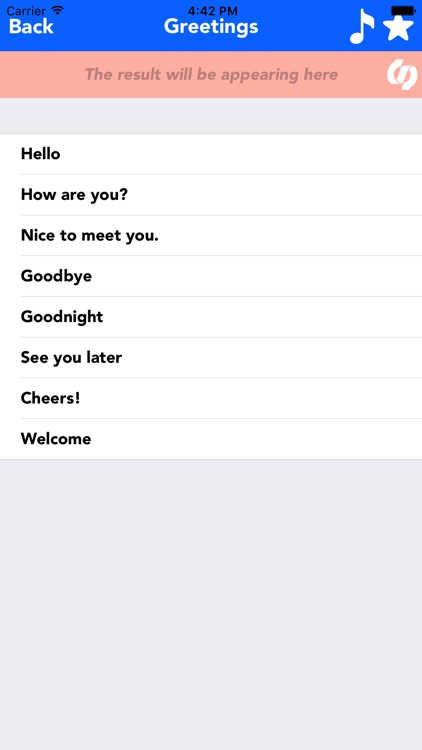A detailed descriptive caption for the given image:

The image showcases a mobile interface of a greetings application, possibly designed for generating automatic greetings. The top of the screen features a blue status bar. On the left corner of the bar, the word "carrier" is visible along with the connection signal icon. Below the blue bar, a secondary bar displays in bold white text, "Back" on the left and a black timestamp reading "4:42 pm" centered. To the right, a white star icon and a musical note are also visible. Following this, a peach-colored section with the light gray text stating "The results will be appearing here" occupies the central part of the screen. Adjacent to this text on the right side, a white ribbon-like icon is observed. Beneath this section, a blank gray bar stretches across the screen, which leads to a list of greeting phrases arranged vertically in bold black text. The phrases include: "Hello," "How are you," "Nice to meet you," "Goodbye," "Goodnight," "See you later," "Cheers," and "Welcome." Concluding the interface, there's another empty gray box at the bottom of the screen.